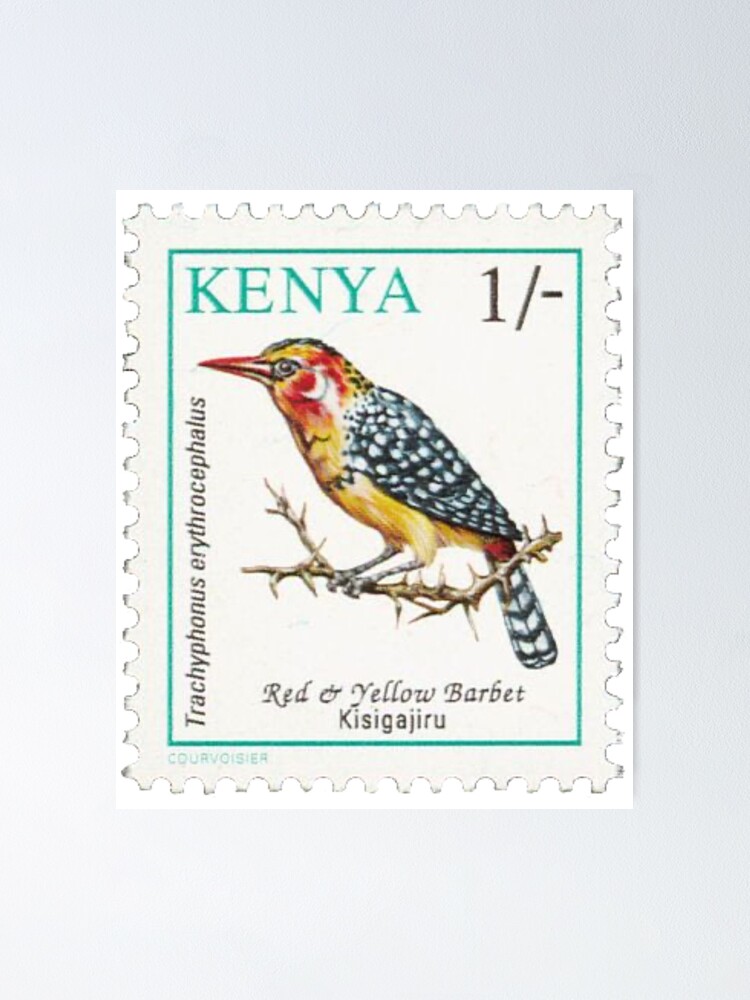The image showcases a brightly lit postage stamp with a detailed and clear design. The stamp features a bird perched on a thorny branch, rendered in vivid colors: black and white speckled tail feathers, a yellow underbody, a red beak, and red accents behind its eyes. The background of the stamp consists of a light blue or grayish-blue hue, bordered by a turquoise-green outline. In the upper left corner, the word "KENYA" is prominently displayed in green capital letters, and just below it, the stamp’s value is indicated by a black "1/-". Along the left side of the stamp, the scientific name "Trachyphonus erythrocephalus" is printed vertically. Below the image of the bird, the common name "Red and Yellow Barbet" is inscribed, along with the name "Kisiga Juru", which could be the local Kenyan name for the bird. The bottom left corner of the stamp also mentions "Corvoisier," possibly the designer or publisher of the stamp.